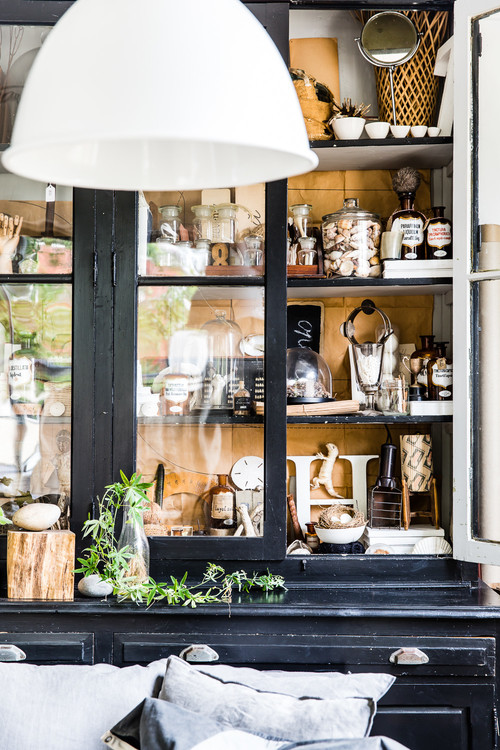The photograph captures a navy blue wooden cabinet with silver handles and glass-paneled doors, situated in a cozy room inside a house. The cabinet doors, particularly the one on the right, are open, revealing four shelves filled with a variety of knickknacks and decor items. 

On the bottom shelf, there is a prominent capital letter 'H' and a glass jar filled with what appears to be rocks or corks. Nearby, a wooden block with an egg shape, and a bottle that might contain medicine sit in close proximity. Moving up, the middle shelves house an assortment of small brown bottles, a cosmetic mirror, and a decor hand, possibly a mannequin hand, along with a decorative number eight. The top shelf features small white vases and more reflective surfaces, likely mirrors.

The foreground of the image displays two or three light blue-grey couch pillows, suggesting the presence of a couch nearby. Adding a vibrant touch, green leaves sprout from a vase on an outside shelf of the cabinet. The color palette of the scene includes black, white, green, tan, brown, and hints of orange.

In the upper left-hand corner, a white light fixture casts a soft glow over the arrangement, while a large white picture adorns the top of the cabinet, further enhancing the decor. The entire setting, captured in portrait view, forms a harmonious mix of colors and textures, accentuating the charm of the room.